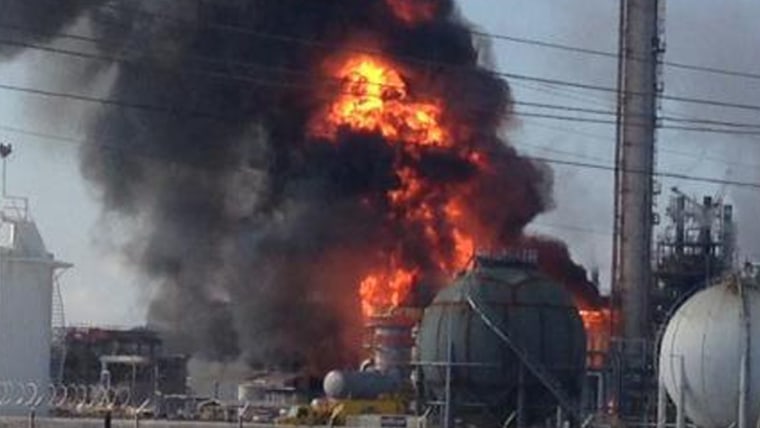This photograph captures a dramatic scene of an explosion at an industrial plant, marked by towering flames and thick, dark smoke billowing into the sky. The image features a variety of industrial structures: at the bottom, a barbed wire fence stretches across the frame, indicating restricted access. To the left, a cylindrical white holding container with an attached staircase stands prominently. Adjacent to it is a larger, green spherical tank with stairs leading to its top, strongly resembling a massive bomb. Right next to it, an almost identical spherical tank is visible, but in white. Rising to the right of these tanks is a giant tower, equipped with a ladder spanning its height, extending out of the frame. Dominating the center and backdrop of the image, the fiery explosion is surrounded by swirling dark gray smoke. Elements such as telephone poles and an additional white tower with a spiral staircase enhance the industrial setting under a blue sky. The entire scene exudes a chaotic and hazardous atmosphere, typical of an industrial disaster.